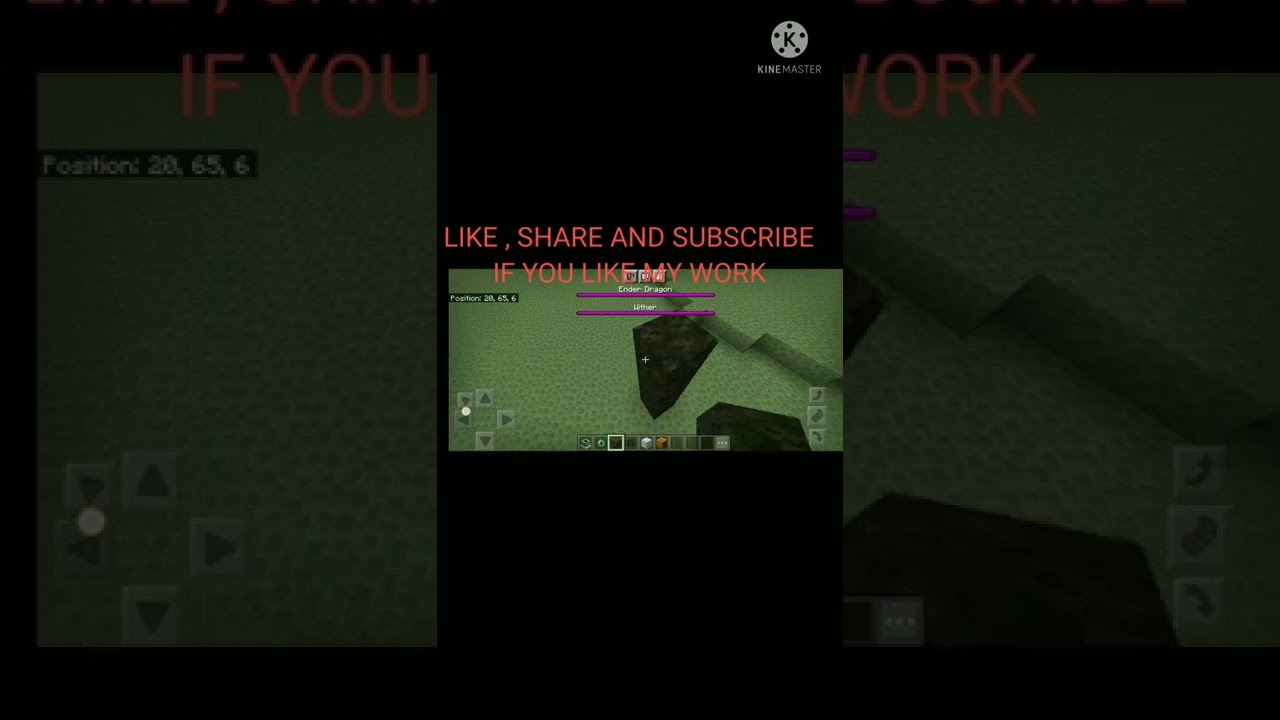The image is a vertical, cell phone-style picture prominently displayed in the center, with a faded, zoomed-in version of the same picture as its background. Both the top and bottom edges of the image include pure black bars that extend fully to the edges. Superimposed over the image, in light red text and divided into two lines, are the words "like, share, and subscribe if you like my work."

The central image appears to be a screenshot from a first-person perspective video game, resembling the mobile version of Minecraft. The environment in the screenshot features green grass and a character's view looking down at a floor made up of three platforms with varying elevations. The HUD (heads-up display) is visible, including a menu area for inventory along the bottom edge, indicating it is gameplay footage. The left and right sides of the screen also have black bars, suggesting that the image is cropped to fit the mobile format. 

There are additional details like a Kinemaster logo in the upper right corner, indicating the use of video editing software. The screenshot captures the game's unique block-building style, and the color palette includes shades of green, black, purple, red, orange, gray, and white. The image seems to be intended for a stream or content promotion, encouraging viewers to support the creator by engaging with their content.